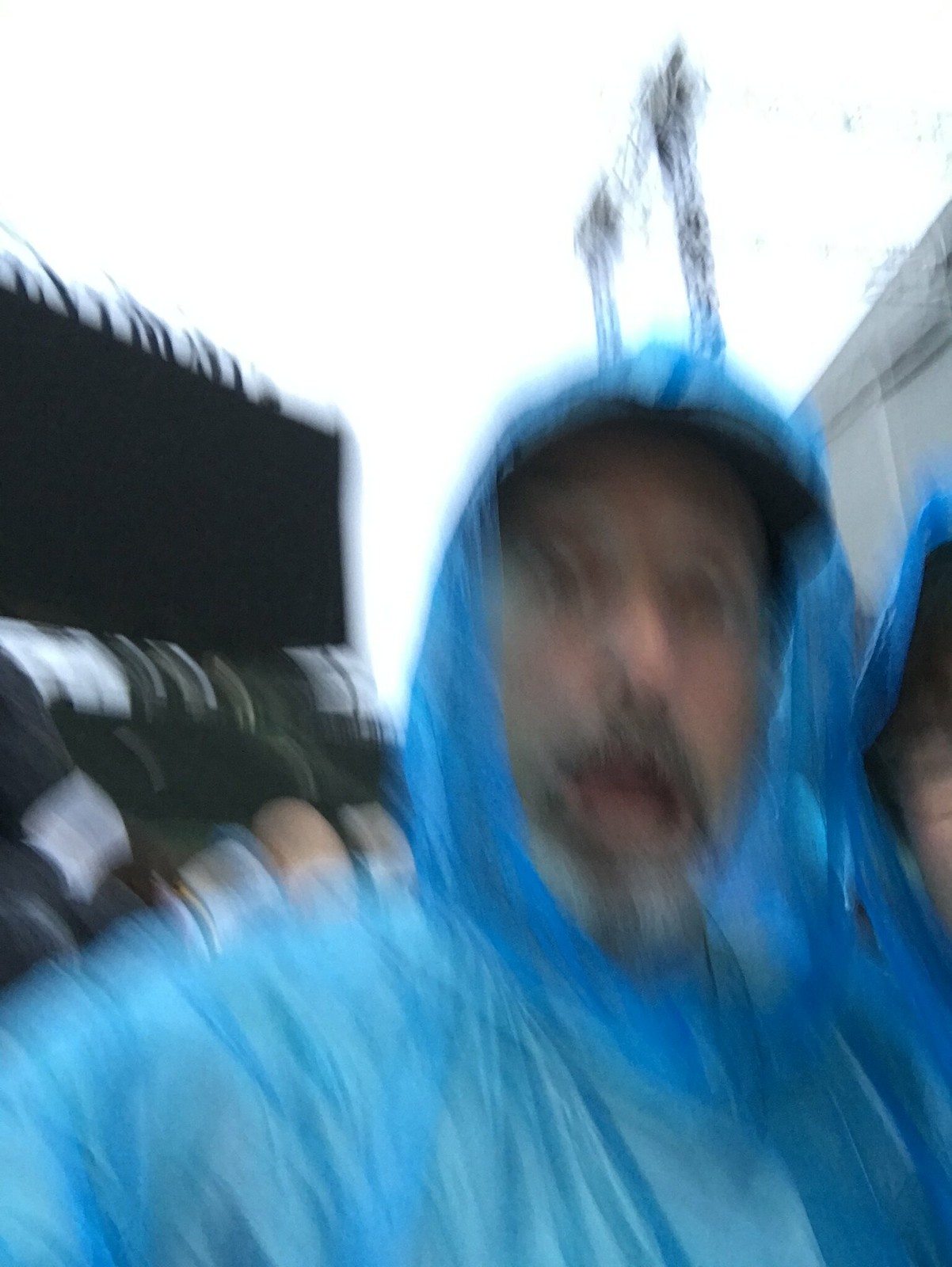In this photograph, an individual captured an extremely close-up shot of a man's face, taken from approximately eight inches away. Due to improper camera settings and possibly a shaky hand, the image is entirely blurred, obscuring finer details. The man's face is the main focus, partly masked by a thin, blue rain poncho typically worn for protection against the rain. Emerging from beneath the poncho are a mustache and beard, subtly visible through the blur. Above his head, the sky is faintly discernible. In the background, there seems to be a black structure with a white awning, although it's not clearly recognizable. Additionally, a white overhead feature—possibly a part of a building—adds to the background elements, though it remains indistinct due to the blurriness of the image.